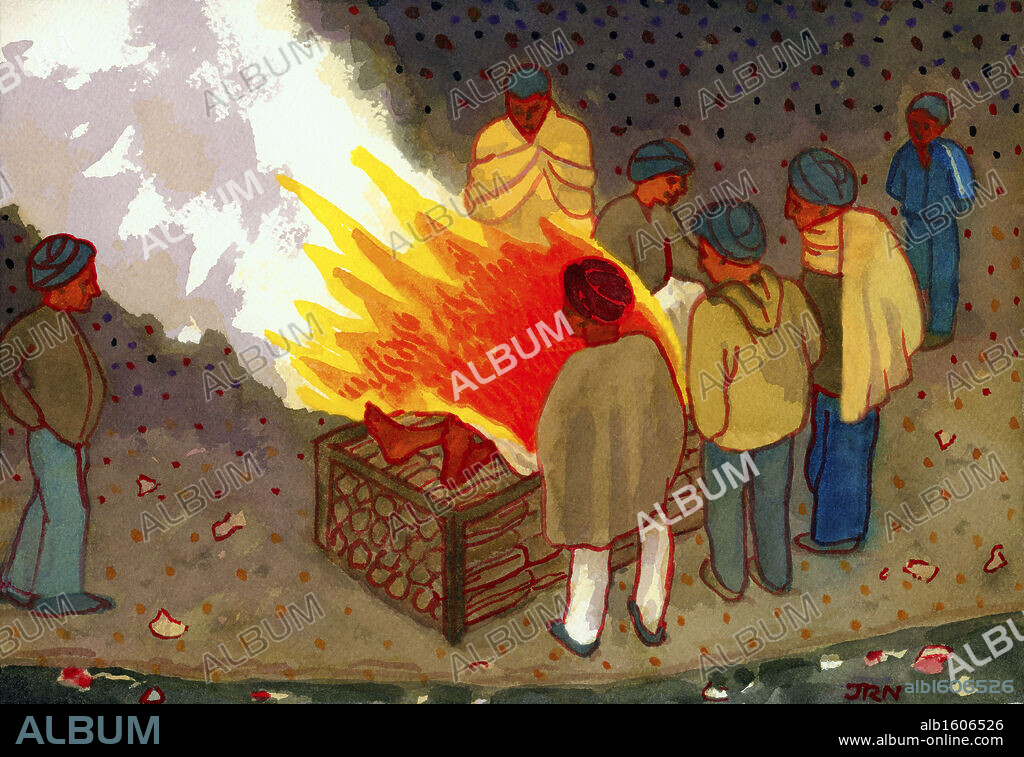The image appears to be a digitally created artwork depicting a ritualistic scene. Central to this illustration is a funeral pyre with flames in vivid hues of red, orange, and yellow, and white smoke billowing to the top left. Surrounding the fire are seven standing figures adorned in various colorful head coverings, predominantly blue and green, with one individual in red. A body, partially shrouded with visible feet sticking out, lies atop the stacked wood, suggesting a ceremonial burning. Overlaying the entire image is a watermark reading "ALBUM" repeatedly, with additional text at the bottom. This includes "album" in blue on the bottom left, and "AIB1606526" alongside "www.album-online.com" in white on the bottom right. The text "JRN" is also placed along the bottom edge. The overall scene, likely an Indian or Pakistani funeral practice, is marked by the somber presence of the individuals and the intense flames of the pyre.